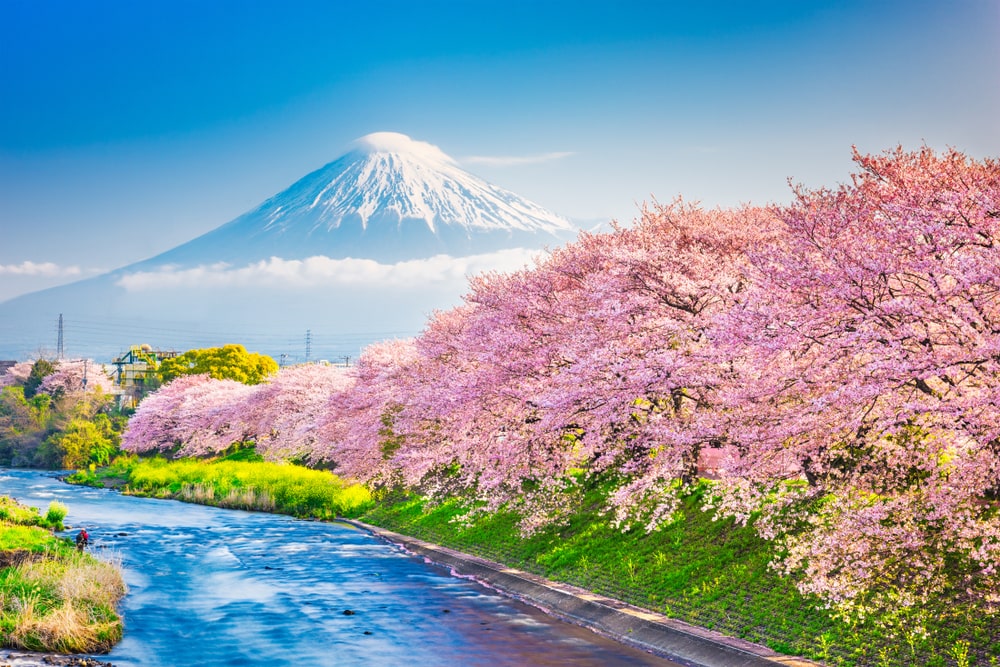This vibrant and striking landscape image could be mistaken for either a painting or a photograph due to its intensity of colors and intricate details. It features a prominent, snow-capped mountain in the distant background, likely Mount Fuji, with a light blue sky and sparse, thin white clouds adorning the upper area of the scene. Swirling, white clouds partially shroud the towering mountain, adding a dramatic sense of height and majesty. 

In the midground, there are distant power lines subtly interwoven into the scenery, bridging the transition between the natural elements and a hint of human presence. Below this, the landscape is dominated by lush vegetation, including bright green grass and bushes. The foreground blossoms with a sea of cherry trees adorned with vivid pink and lilac flowers, creating an overwhelming explosion of color. These cherry blossoms extend over a green flower bed that sits adjacent to a paved pathway.

Notably, a river flows through the lower part of the scene, beginning at the lower left corner and meandering towards the bottom center, its origin and destination left to the imagination, adding to the enigmatic beauty of the image. The harmonious combination of natural elements and varying hues makes this scene extraordinarily picturesque and immersive.